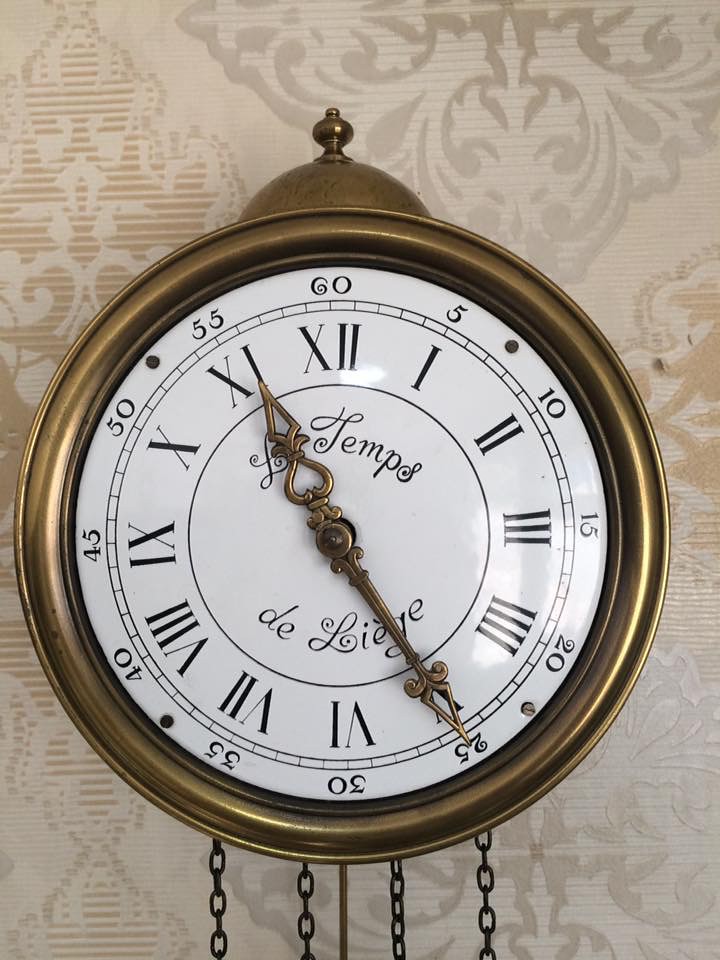This close-up image showcases a vintage gold clock mounted on a wall adorned with a faded fleur-de-lis patterned wallpaper in shades of gray, silver, and bronze. The ornate, round clock features a semi-circular decorative crown at the top, reminiscent of a pocket watch, crowned with a spindle. The clock face is white, encased in a gold rim, further bordered by a black trim. It displays elegant, ornate gold hands. Surrounding the center circle, "Les Temps" is written in cursive black script at the top, and "Des Lièges" at the bottom. The inner circle displays Roman numerals, while the outer edge marks traditional minute intervals in Arabic numerals from 5 to 60. Four gold chains, potentially with weights, hang down from the bottom of the clock, adding to its vintage charm and intricate design.